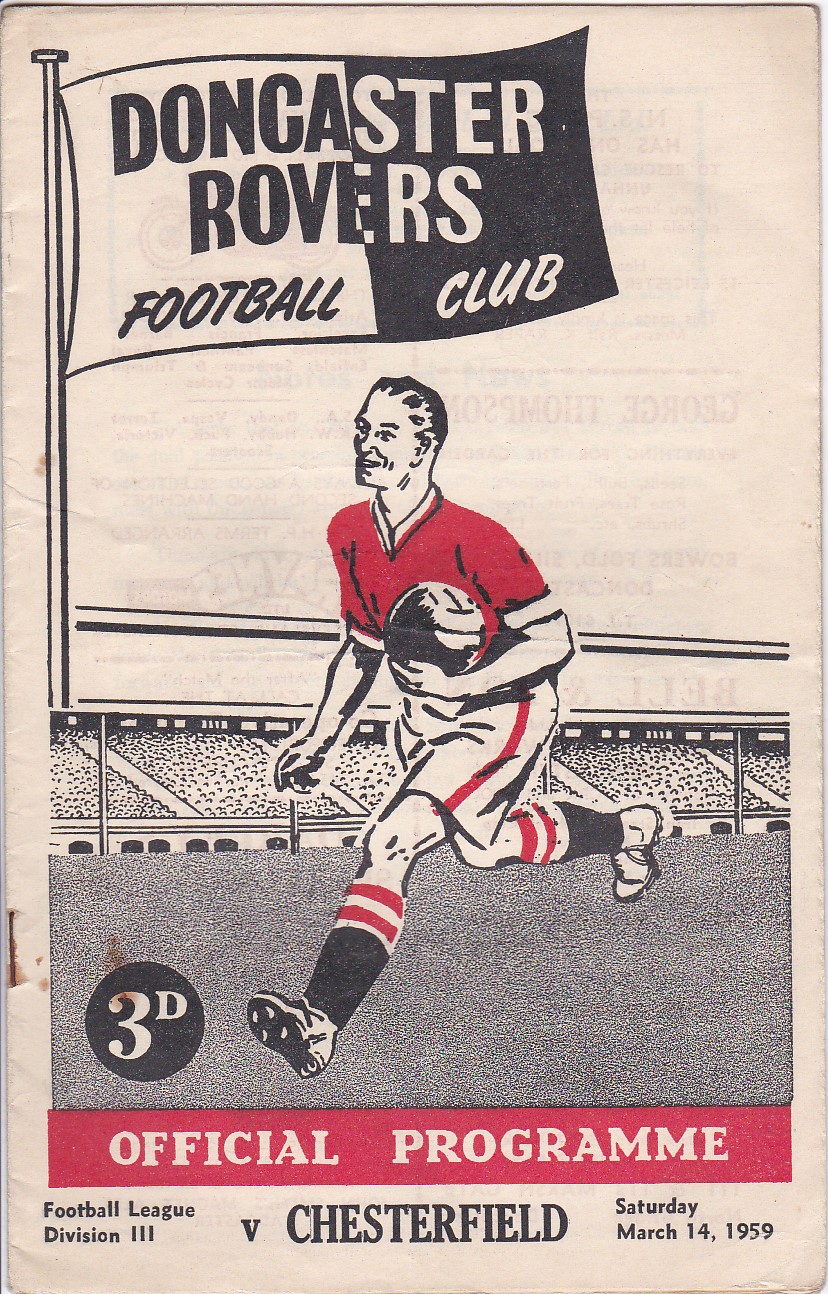This image depicts the hand-drawn cover of an official program for the Doncaster Rovers Football Club. The background paper has aged to a beige or cream color. The central illustration features a soccer player in a red T-shirt, white shorts with a red stripe down the sides, and white socks with two red bands. He is depicted running on the field, holding a soccer ball, with a stadium visible in the background. To the right, there is a flag with "Doncaster Rovers Football Club" written on it; the flag is divided with one half white with black lettering and the other half black with white lettering. At the bottom of the cover, the text reads: "Official Program, Football League Division 3 vs. Chesterfield, Saturday, March 14th, 1959." This cover suggests that the club match took place on that date. A small black circle marked with "3D" is also visible, likely indicating the program's price.